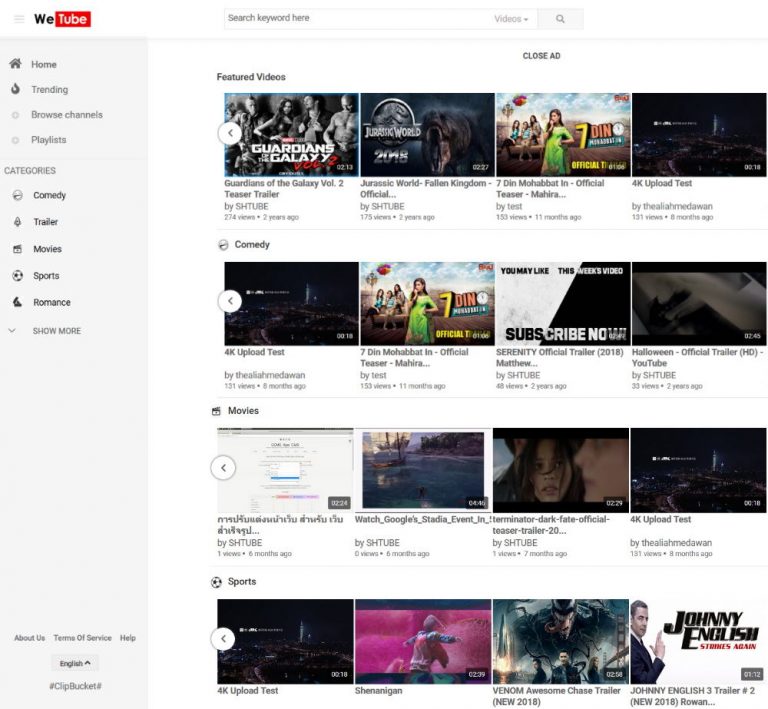The image appears to be a screenshot of the Weetube website interface. At the top, the Weetube logo is displayed prominently, featuring the letters "WE" in black, followed by a horizontally extended red rectangle containing the word "tube" in white. Below the logo, a vertical gray sidebar runs down the left side, featuring navigation options in black text: "Home," "Trending," "Browse Channels," and "Playlists." Further down, under a barely visible gray line, the sidebar lists "Categories" in gray, with subcategories such as "Comedy," "Trailer," "Movies," "Sports," "Romance," and a "Show more" option with a drop-down menu.

In the central area of the page, at the top, there's a search bar with the text "Search keyword here," accompanied by a drop-down menu labeled "Videos" and a gray button with a search icon on the right side. Below another gray line, the section for featured videos is showcased, displaying four videos in a horizontal row. The featured videos include: "Guardians of the Galaxy Volume 2 Teaser Trailer," "Jurassic World: Fallen Kingdom Official Trailer," "7 Din Mohabbat In Official Teaser," and "4K Upload Test."

Following the featured section, the "Comedy" category is highlighted, presenting four videos in a row: "4K Upload Test," "7 Din Mohabbat In," "Serenity Official Trailer (2018, Matthew)," and "Halloween Official Trailer HD YouTube."